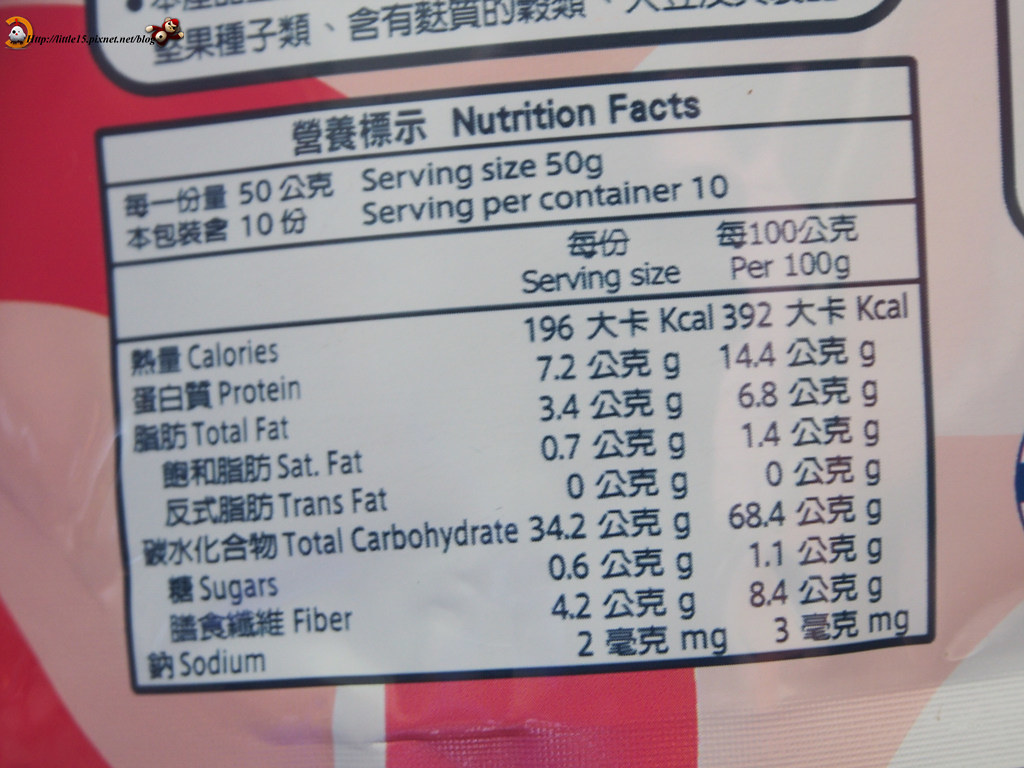The image features a detailed nutrition facts label accompanied by Chinese calligraphy. On the left side of the nutrition facts panel, the serving size is listed as 50 grams in blue text, with servings per container marked as 10. Below this, the serving size is once again specified, followed by Chinese script and the notation "per 100 grams." The label further breaks down nutritional components such as calories, protein, fat, saturated fat, trans fat, carbohydrates, sugars, fiber, and sodium. Specifically, it indicates that per 100 grams, the item contains 196 calories, 7.2 grams of protein, 3.4 grams of fat, 0 grams of trans fat, 2 grams of sodium, 0.6 grams of sugars, and 4.2 grams of fiber.